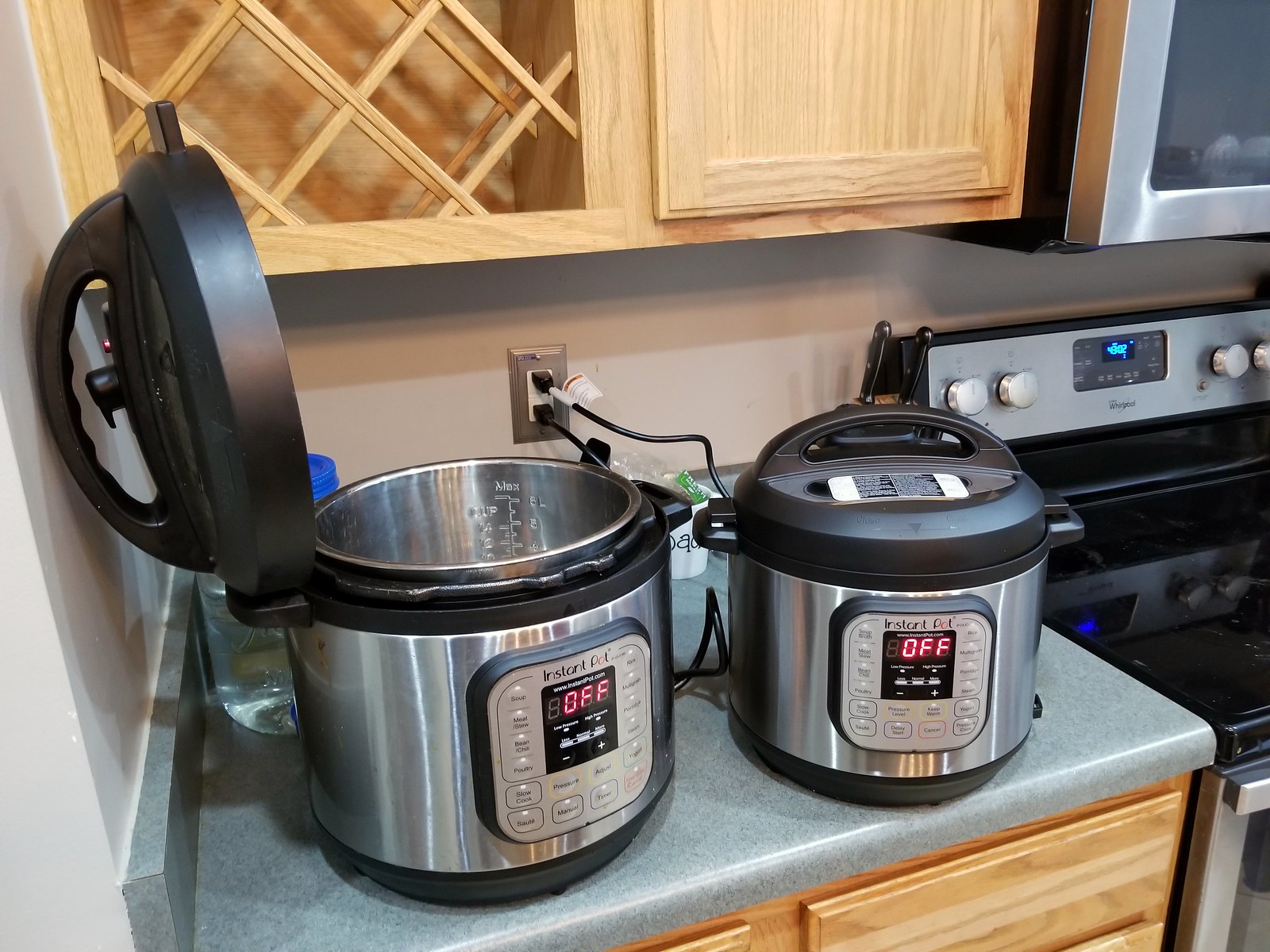The color photograph captures a cozy corner of a kitchen, where two relatively new Instant Pots are positioned on a small, almost green countertop next to a stainless steel stove with a black top. Both Instant Pots, which are plugged into a nearby outlet, display the word "OFF" in red and appear to be functional but not currently in use. One of the Instant Pots has its lid open, revealing an empty interior. Above the countertop, light wooden cabinets with a crisscross design on the glass doors provide a quaint storage solution. The stove's control panel includes a small blue clock that is discernible but too small to read clearly, adding a subtle touch of modernity to the kitchen's warm and inviting atmosphere.